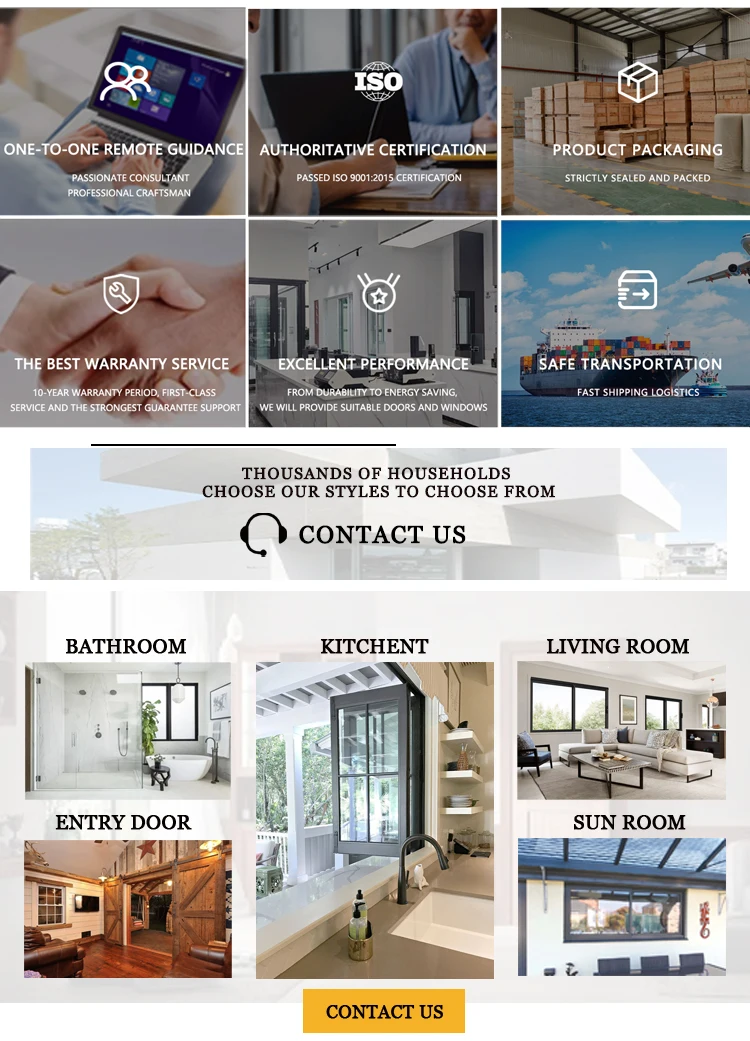This image showcases an advertisement for an interior decorating service. It consists of a series of photographs accompanied by descriptive text, organized into two main sections.

At the top, there are six images arranged in two rows of three, each with white text overlay:
1. An image of a laptop with the text "One-to-One Remote Guidance."
2. Two people working at a table with a laptop, labeled "Authoritative Certification."
3. A warehouse filled with boxes, captioned "Product Packaging."
4. Two individuals shaking hands, accompanied by the words "Best Warranty Service."
5. An office space with the phrase "Excellent Performance."
6. A shipping container being transported, labeled "Safe Transportation."

In the center, there is black text that reads: "Thousands of Households Choose Our Styles." Accompanying this text is a headset icon and the words "Contact Us."

Below this central text, there are five additional photographs, each with a black text label:
1. A photograph of a bathroom labeled "Bathroom."
2. A living space featuring barn doors, labeled "Entry Door."
3. A kitchen counter and open windows, with the label "Kitchet" (a misspelling of "Kitchen").
4. A living room labeled "Living Room."
5. A sunroom labeled "Sunroom."

Each element of the advertisement is designed to emphasize different aspects of the interior decorating service, from remote guidance and certification to product packaging, warranty service, performance, and transportation.